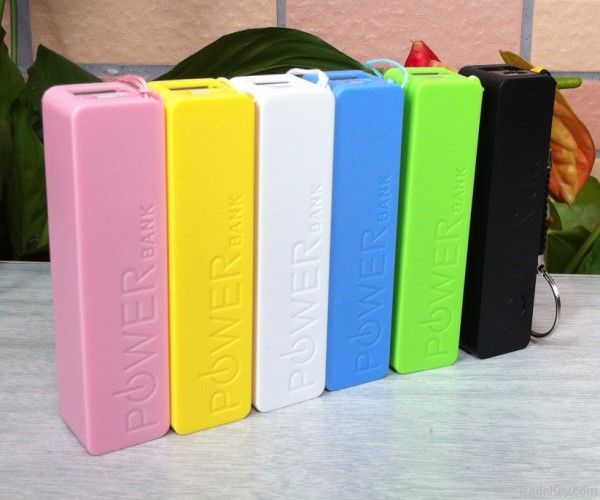The image depicts six vertical, rectangular power banks for charging cell phones or tablets. They come in an array of vibrant colors: pink, yellow, white, blue, lime green, and black. Each power bank features the words "power bank" imprinted on its neoprene-like outer layer and includes a matching colored wrist strap with a metal ring loop for easy carrying. They are lined up from left to right on a light gray surface, possibly a marble or Formica countertop. In the background, there is a wall with pink tiles and silhouettes of foliage, adding a touch of nature to the scene.